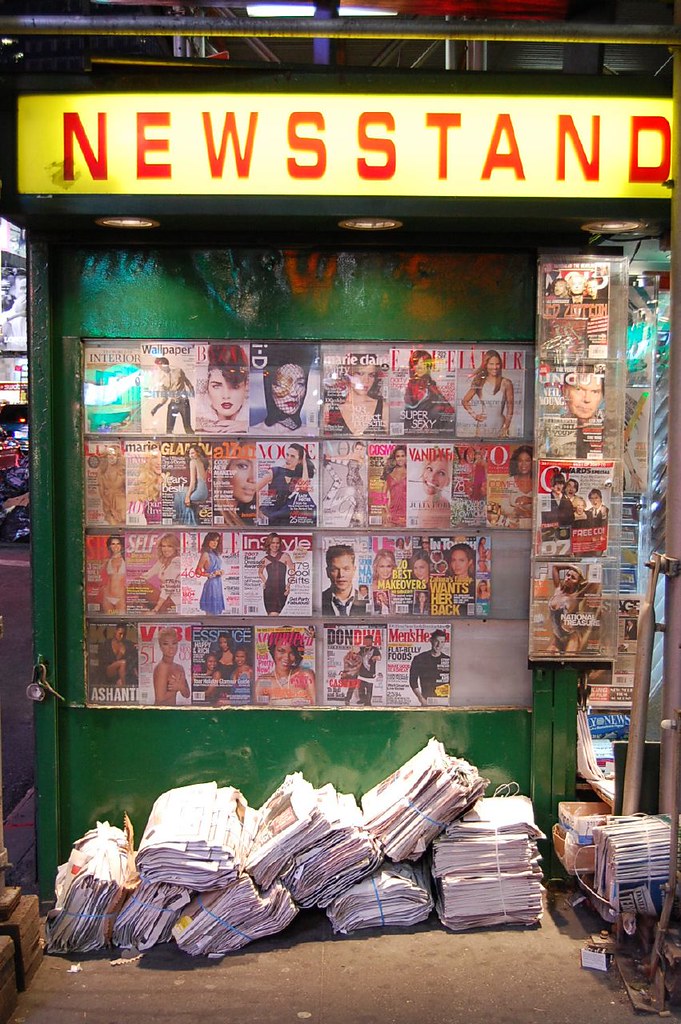This is a detailed color photograph of a busy city newsstand, likely in New York, encapsulating the vibrance and variety within its green walls. The newsstand features a prominent, illuminated yellow sign with the word "newsstand" emblazoned in red letters. Below it, three overhead can lights cast a soft glow onto the scene. Numerous colorful magazines are meticulously arranged in four rows both at the center and right sections of the display, visible through a plexiglass window. Titles such as Glamour, Marie Claire, InStyle, Self, Don Diva, Men's Health, Vibe, Essence, Uncut, and a magazine featuring Led Zeppelin can be identified among others. The ground in front of the kiosk is a rough, gray concrete, scattered with bundles of newspapers bound in blue or white plastic straps. Silver metal poles frame the sides of the structure, and a lock is noticeable at the lower left corner, safeguarding the eclectic collection of periodicals. To the left, hints of a bustling city environment emerge, including piled garbage bags in the center view, enhancing the urban atmosphere of this quintessential newsstand.